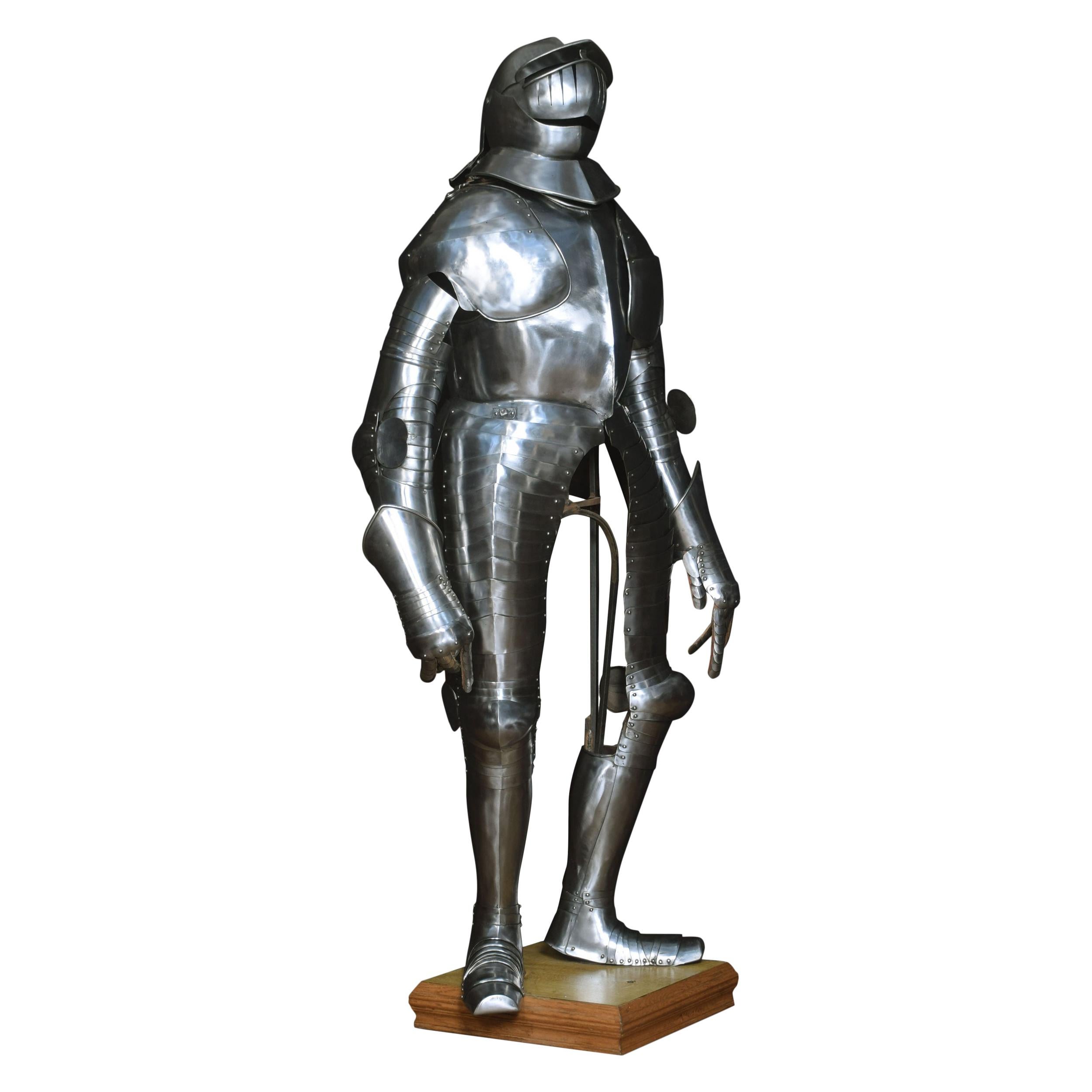The image portrays a detailed display of a knight's armor mounted on a brown wooden pedestal with a subtle orange hue. The armor, which is predominantly silver with black shadings, stands in a poised position with the left foot halfway off the pedestal and the tip of the right foot slightly overhanging. The fully enclosed helmet seamlessly connects to the muscular contours of the chest plate, which extends protectively across the entire body, down to the articulated fingers on both sides. The background is stark white, suggesting either a plain photographic backdrop or a digitally created scene. The left leg of the armor (on the image's right side) seems incomplete, missing a portion and revealing a vertical brown bar. The armor's mask is down, and the arms rest at the sides.